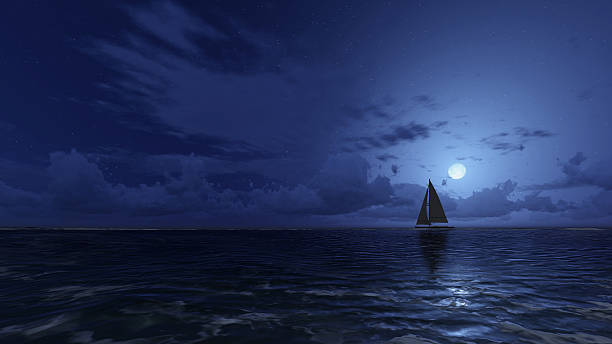In this nocturnal landscape photograph, a large sailboat with both sails open is captured near the horizon, seemingly adrift on a vast and dark water body, either a sea or a lake, under a rich, dark blue sky. The sailboat, illuminated faintly by moonlight, appears almost as a silhouette. The full moon, positioned just above the water to the right of the sailboat, casts a glowing reflection on the rippling waves below. The tranquil night scene is accented by wispy, streaky clouds higher up and a few fluffy, flat-bottomed clouds closer to the horizon. The expansive sky, devoid of stars, and the gentle movement of waves enhance the serene ambiance of this moonlit seascape. No land or people are visible, emphasizing the solitary beauty of the boat under the vast, dark canopy.